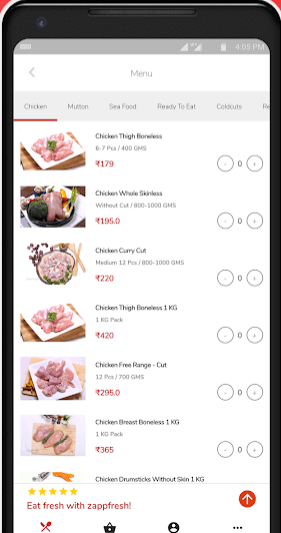In the image, a smartphone displays an open food-ordering app, captured from a slight angle that showcases the phone's frame and bezels against a neutral background. The app interface features a predominantly white background, prominently displaying the word "Menu" at the top, indicating that the user is currently navigating through the chicken section of the app. Various cuts of chicken are listed, each accompanied by small-sized text that reads descriptions like "Chicken Free Range Cut," "Chicken Breast Boneless," and "Chicken Thigh Boneless," among others. The images of the chicken cuts are paired with prices in an unfamiliar currency. At the bottom of the phone screen, a promotional banner with five stars and the phrase "Eat Fresh with Zap Fresh" highlights the app's branding. Additionally, navigation icons are visible, including a shopping bag or basket symbol and a profile section, hinting at other functionalities available within the app. This detailed composition suggests the app serves as a digital marketplace, likely for a supermarket or specialized poultry store.